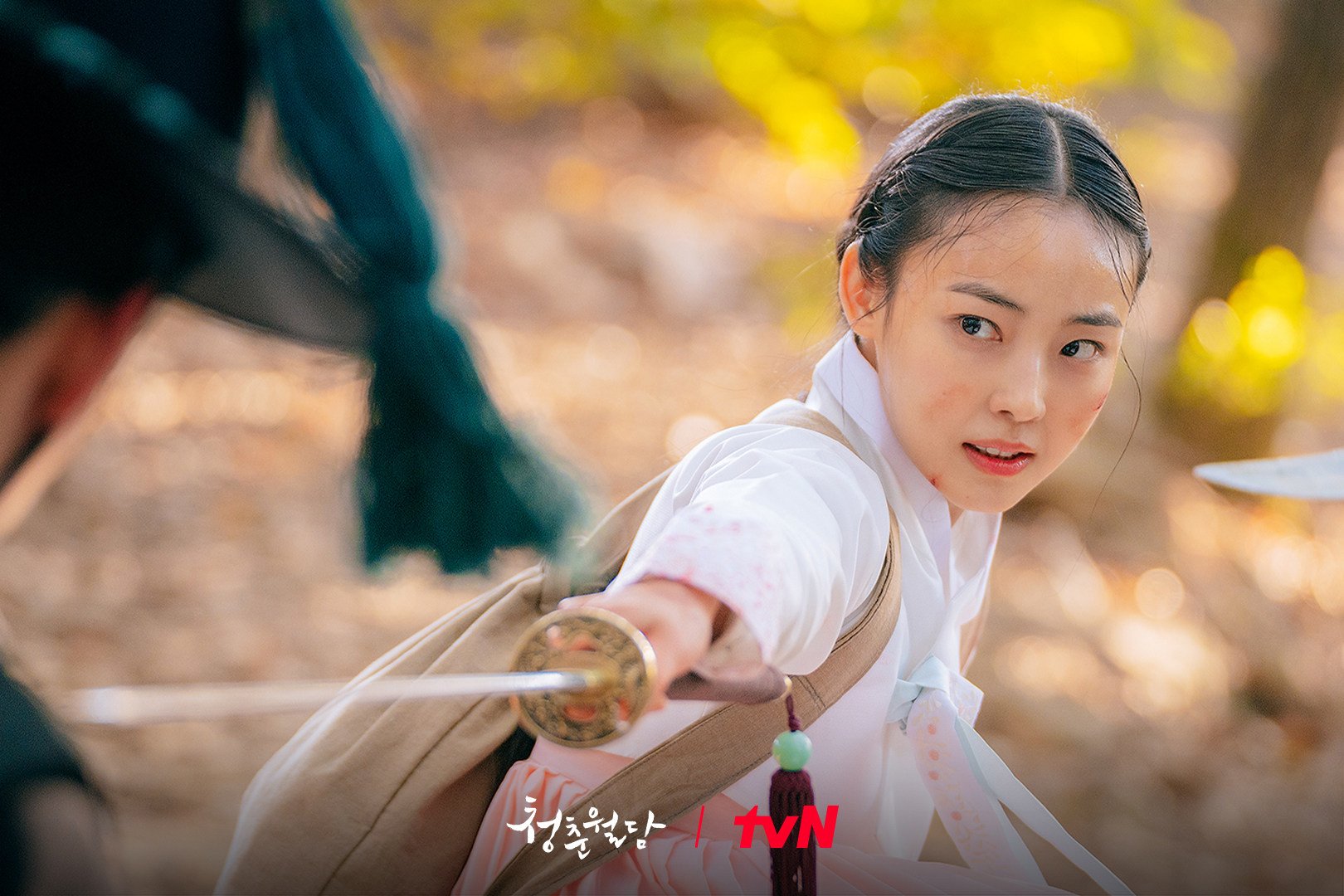In this striking image, we see an Asian girl, likely aged around 15 or 16, engaged in a tense sword fight, exuding a mix of fear and confidence. Dressed in a white outfit with a hint of pink around her waist, she brandishes a striking sword with a golden handle and a silver blade. Her dark hair, parted down the middle, has delicate wisps framing her face, which bears a smudge of what appears to be blood, highlighting the intensity of the confrontation. The scene has a backdrop of woods with yellow lights or foliage subtly visible, suggesting an outdoor setting. The photo, which could be a movie still, has the TVN logo in red at the bottom and some Asian script, possibly Korean, nearby. The girl's direct focus contrasts with the partial glimpse of a soldier opponent, identifiable by just an ear, some hair, a hat, and shoulder armor. The tension and narrative embedded in this image are palpable, making it an evocative portrayal of determination and conflict.